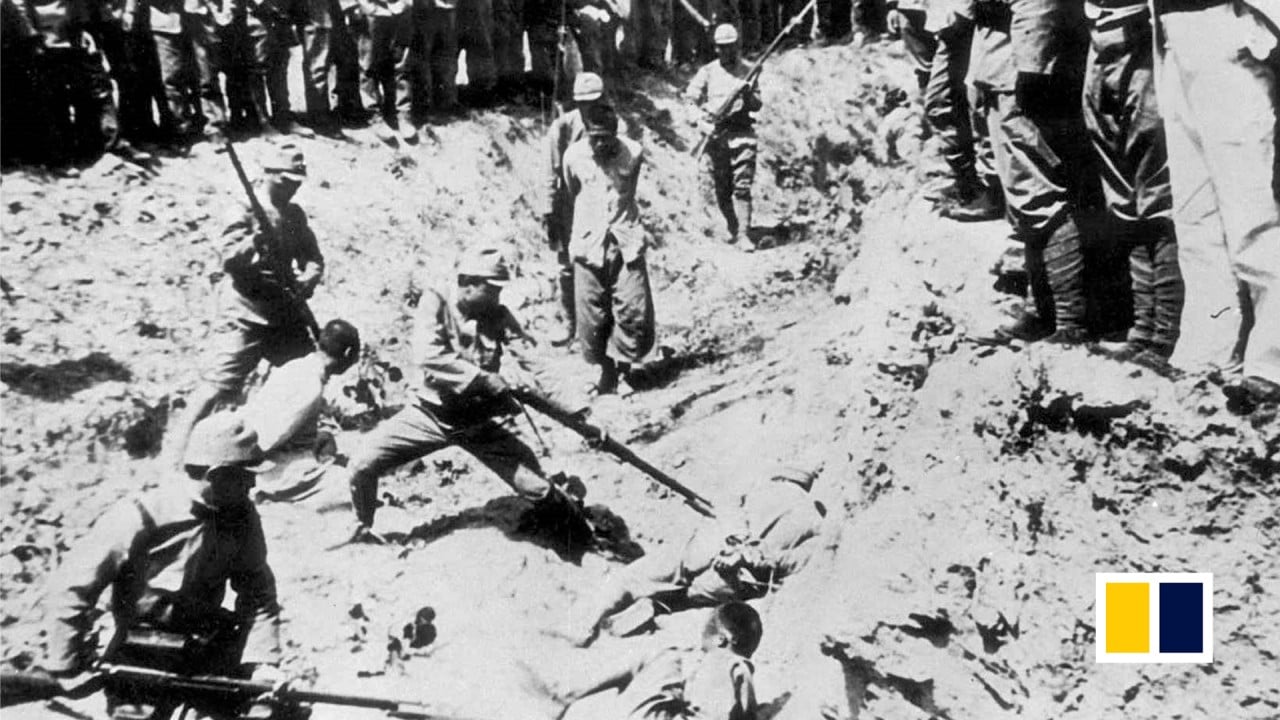The black and white photograph captures a haunting historical scene of violence and death, likely during wartime. It depicts a freshly dug trench where prisoners, possibly of Asian descent, are confined with their hands tied behind their backs. The scene is rife with tension and brutality, as soldiers, who appear to be Japanese, stand around the edges of the trench, brandishing rifles and bayonets. Central to the image is a soldier seemingly in the act of either stabbing or shooting a prisoner who lies on the ground, a moment frozen in grim clarity. The prisoners wear simple, hatless garments, contrasting with the soldiers' uniforms and small-brimmed hats. Spectators with somber expressions line the ditch's periphery, their legs visible at the trench's edge. In the lower right corner of the image, a yellow and black flag with a white border can be seen, adding an odd splash of color to the monochrome devastation. The ground, disrupted and uneven, speaks to the trench's hasty excavation, destined to serve as an open grave for the unfortunate souls within.